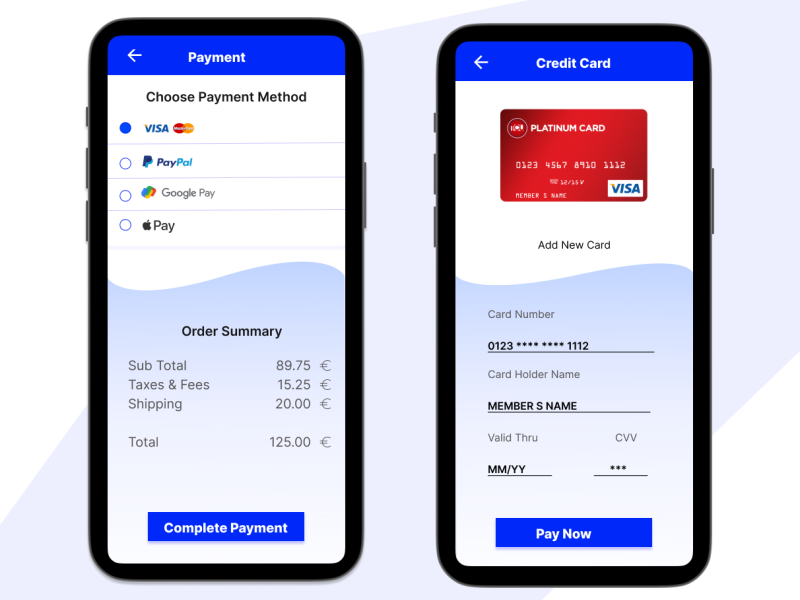The image showcases a two-step online payment process.

**Step 1: Payment Method Selection**
- At the top, a blue banner prominently reads "Payment."
- Below this, the text "Choose Payment Method" is displayed in black letters.
- Available payment options include Visa, PayPal, Google Pay, and Apple Pay, each represented by their respective logos.
- An order summary is presented:
  - Subtotal: €89.75
  - Taxes and Fees: €15.25
  - Shipping: €20.00
  - Total: €125.00
- A blue rectangular button at the bottom prompts users to "Complete Payment."

**Step 2: Credit Card Information**
- The second page also features a blue banner at the top, now labeled "Credit Card" with a white arrow pointing to the left.
- Below, there's the image of a red platinum card showcasing the digits "0123 4567 8901 112." The card has an expiration date of "12/25."
- Fields for adding card details include:
  - Card Number
  - Member's Name
  - Valid Through
  - CBB (Card Verification Code)
- At the bottom, another blue rectangular button reads "Pay Now."

This detailed progression through the payment interface provides a user-friendly and visually organized system for completing online transactions.